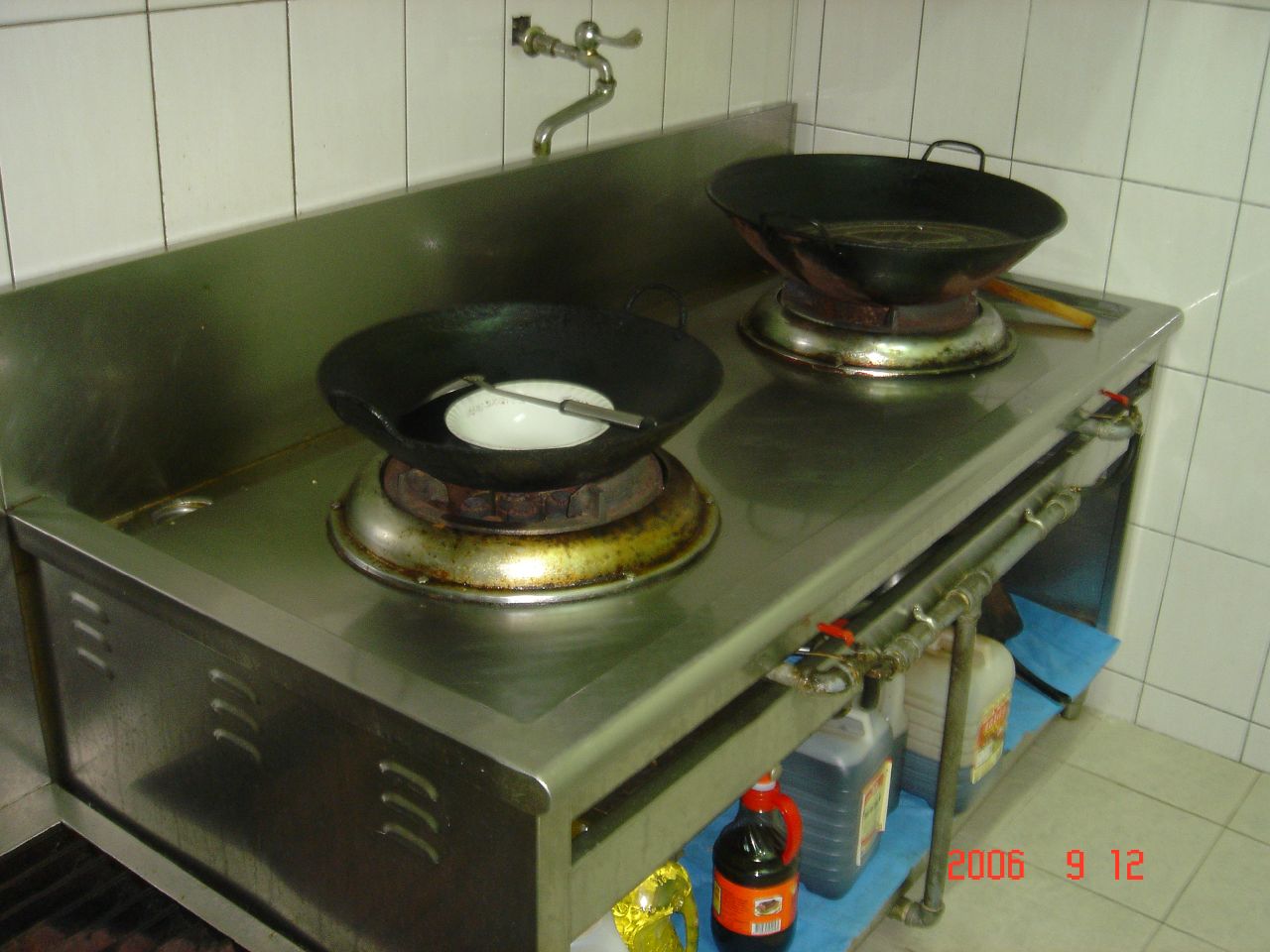This photograph, taken on September 12, 2006, captures a commercial cooktop situated in the left corner of a room with white square tiles and dark grout on the walls and floor. The older, silver stove features a long rectangular top with two large woks, each sitting on a cylinder-type burner. One wok contains a white cylindrical object and a silver stirring instrument laid face down. A tube with a gas control handle extends from the back of the stove into the wall. Below the stove, on a shelf, are multiple containers: a tall, thin bottle with a red label and pouring handle, two large plastic jugs (one three-quarters empty), another container filled with black items, and an additional fabric-covered item. The setting and equipment suggest a commercial kitchen environment.